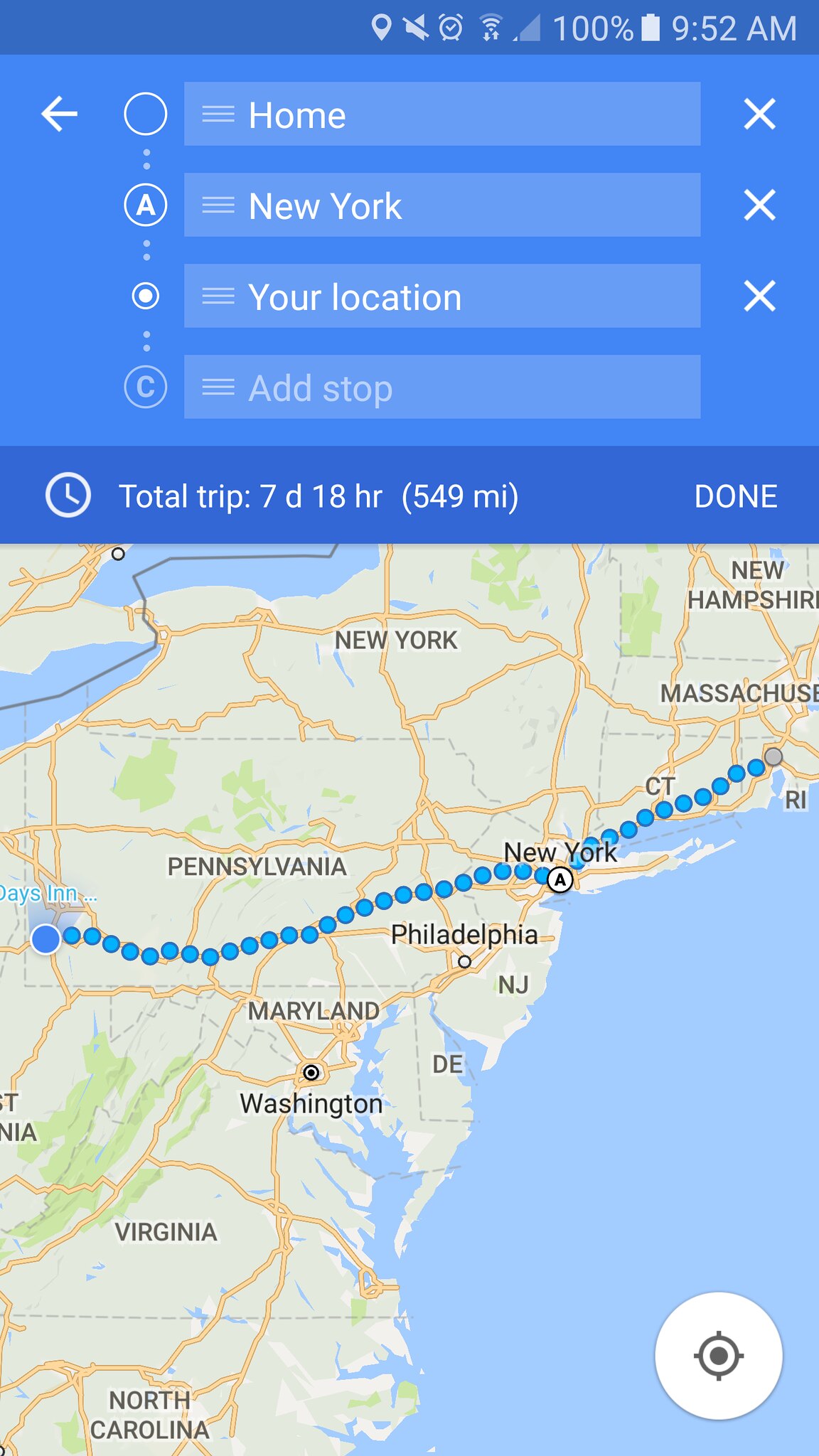This image is a screenshot of Google Maps on a phone, capturing a detailed route plan. At the top, a dark blue strip displays various icons such as a location icon, a silent mode indicator, an alarm, and a signal bar showing just one bar. The battery is fully charged at 100%, and the time displayed is 9:52 AM. Below this, a lighter blue box highlights the route details: the origin point is set to 'Home,' and the destination is New York, with no additional stops.

In the main portion of the screen, a map shows a blue dotted route originating from the middle of Massachusetts, traversing through New York, and extending through Pennsylvania to the Ohio border. The map encompasses an extensive region from New Hampshire down to North Carolina, with states like West Virginia, Virginia, Washington, D.C., and Maryland also visible. The dotted line indicates a total trip duration of 7 days and 18 hours, covering a distance of 549 miles, which suggests it may represent a walking route.

Additional elements include a back arrow and cancel options for editing the route, a clock icon at the bottom indicating the trip details, and a small compass in the bottom left corner. The map itself is color-coded with tan for land, orange for borders, and green patches, likely representing parks or less developed areas. The Atlantic Ocean and some of the Great Lakes are also visible on the map, adding geographic context to the route's extensive coverage of the northeastern United States.